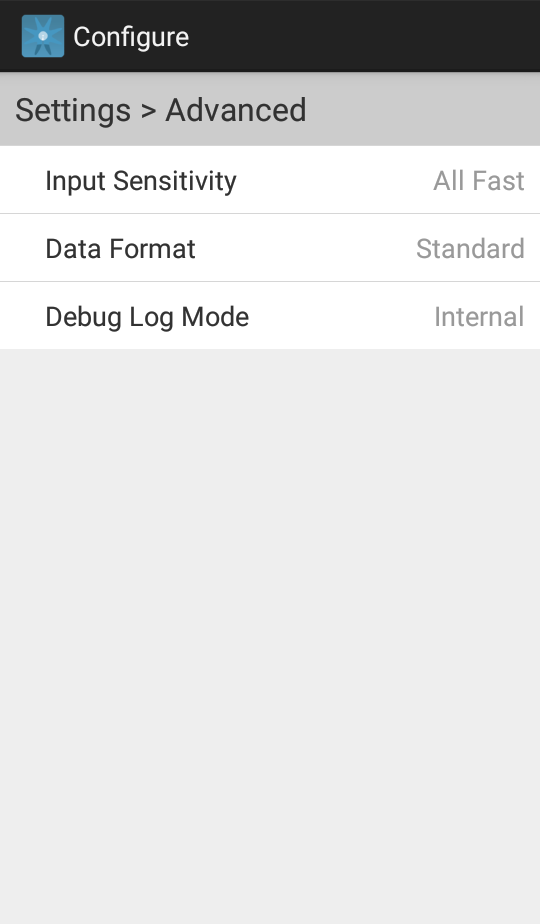The image depicts a screenshot from a cell phone displaying a configuration page. At the top, within a black rectangular banner, the word "Configure" is prominently displayed in white letters. Adjacent to this text is a teal square icon featuring a white circle with a floral design.

Beneath this banner, the background transitions to gray, displaying several options. The first section is labeled "Settings" and includes a right-pointing arrow next to the word "Advanced." Below, the interface is divided into three elongated, narrow rectangles separated by faint gray lines.

The first rectangle is labeled "Input Sensitivity" in black print, and at the far right of this row, it reads "All Fast." The second rectangle is labeled "Data Format" in black print, with "Standard" stated at the far right. The third and final rectangle is marked "Debug Log Mode" in black print, indicating "Internal" in gray print at the far right. The bottom of the screen is completed with a solid gray rectangle.